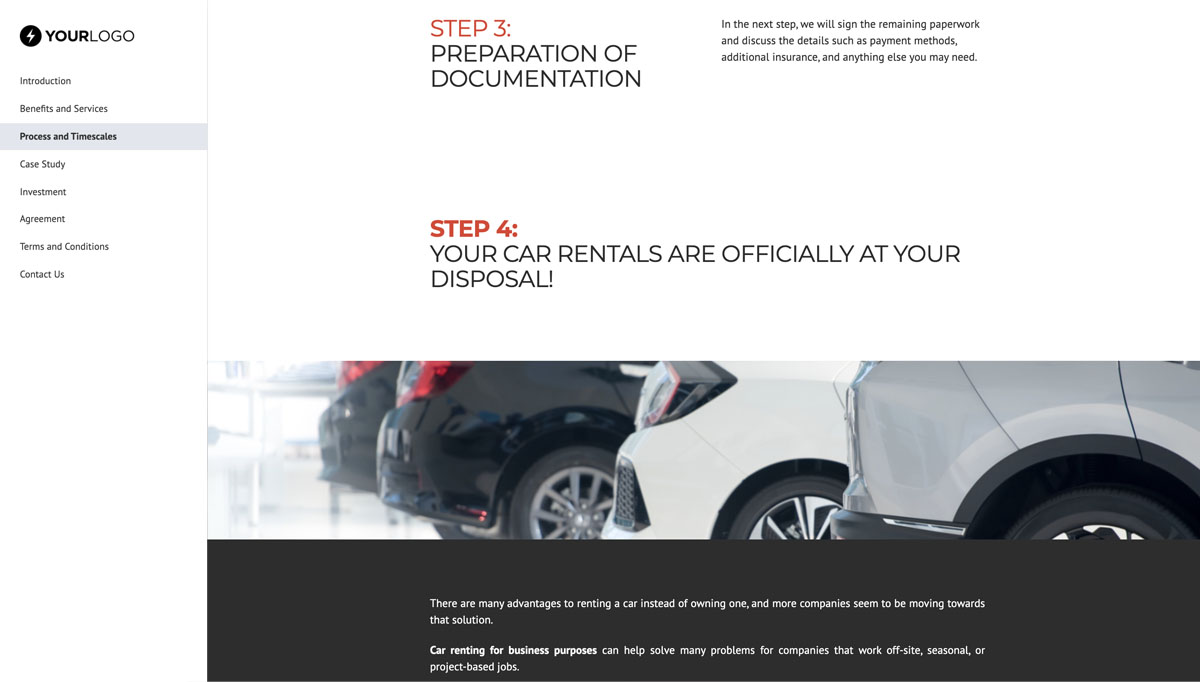The image depicts a secondary webpage of a logo creation service website. The top left corner features the service's logo, a black circle adorned with a subtle white lightning bolt. Below the logo, navigation categories are listed, including "Introduction," "Benefits and Services," "Process," "Case Study," "Agreement," "Terms and Conditions," and "Contact Us."

The page is specifically identified as "Step 3: Preparation of Documentation" in a multi-step process. A note clarifies, "In the next step we will sign the remaining paperwork and discuss details such as payment methods, additional insurance, and any other needs."

Step 4 is prominently mentioned, noting that "your car rentals are officially at your disposal." Accompanying this is an image of several parked cars, viewed from the rear. The cars, parked diagonally, include a gray vehicle, a white vehicle, and two black vehicles.

Below the car image, a black box contains text highlighting the benefits of renting a car over owning one, noting an increasing trend among companies towards car rentals. Additional explanatory text follows beneath this initial statement.